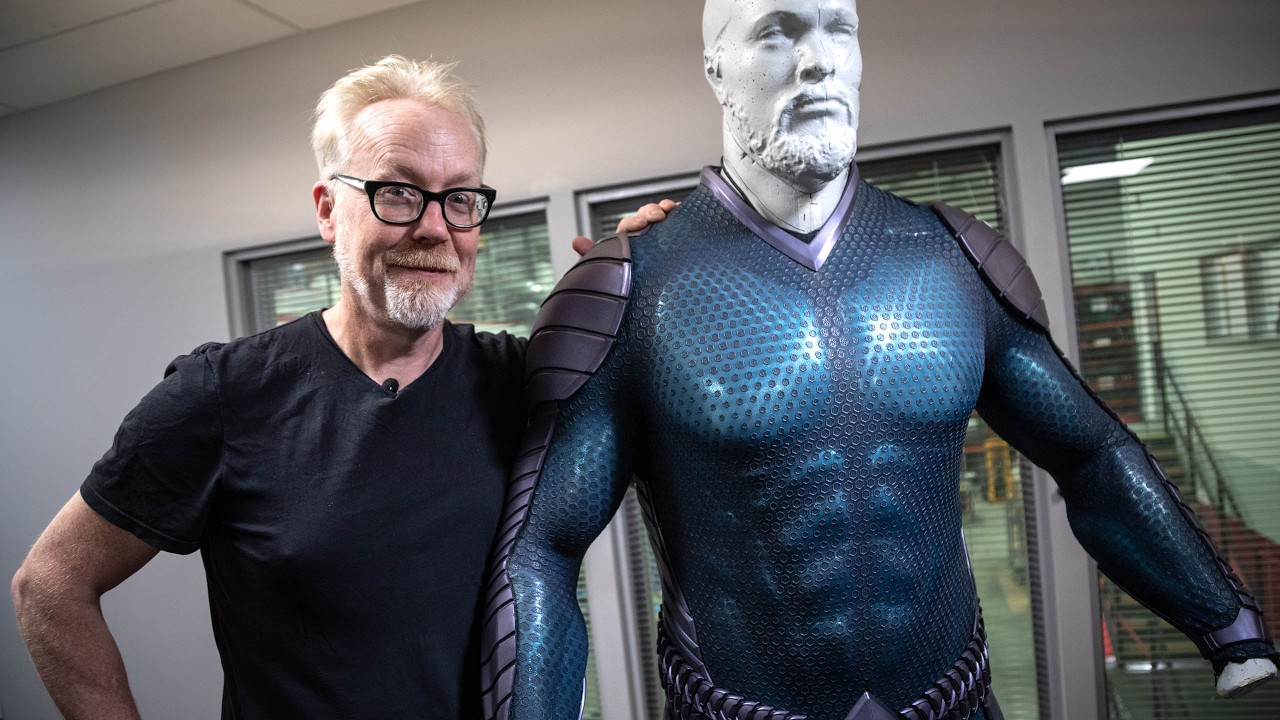In this horizontally aligned rectangular photograph, an older man, likely in his 50s or 60s, stands inside a room with light gray walls and a white-tiled ceiling. Behind him are three vertical rectangular windows fitted with mini blinds that reveal another room beyond. The man, smiling with a closed mouth, has short blondish-white hair, a matching mustache, and beard, and wears black-rimmed glasses. Dressed in a short-sleeved black t-shirt, he poses with his right hand on his hip, while his left arm rests on a shoulder of a nearby sculpture.

The sculpture, detailed and high-quality, appears to be a formidable superhero-like figure. It is adorned with a textured, black, and metallic costume that showcases a muscular chest and defined abs. The attire includes darker metallic shoulder pads and arm padding, and it features long sleeves with a scaly appearance, as well as a silverish belt. The face of the sculpture, carved from a light gray-colored stone, presents a robust appearance with a full beard and mustache, yet remains unpainted, highlighting its raw stone finish.